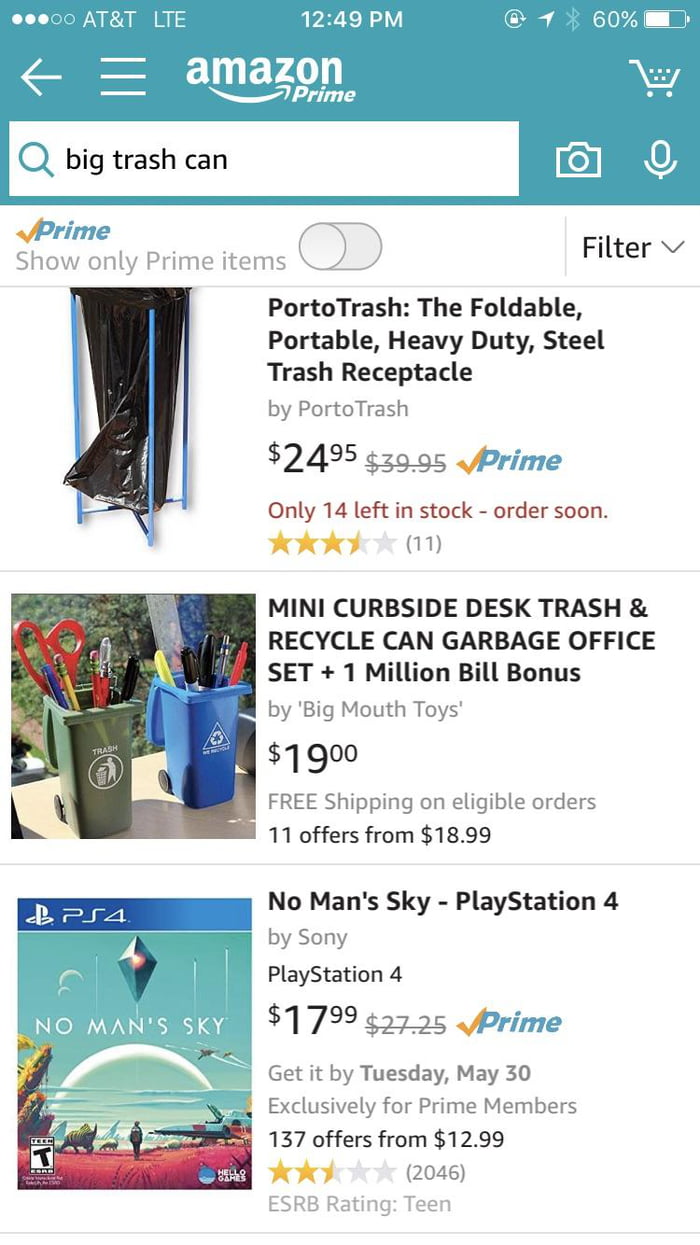Caption: The image is a screenshot from Amazon Prime displaying search results for “Big Trash Can.” The first item featured is the "Porto Trash Foldable Portable Heavy Duty Steel Trash Receptacle" priced at $24.95 with Prime delivery, highlighting that only 14 units are left in stock and urging customers to order soon. This product has 11 reviews and includes a picture of a black trash bag supported by a sturdy steel stand. The second item is the "Mini Curbside Desk Trash and Recycle Can Garbage Office Set Plus 1 Million Bill Bonus" by Big Mouth Toys, available for $19.00 with free shipping on eligible orders and 11 offers starting at $18.99. The accompanying image shows two small desk trash cans: a green one filled with red scissors, pencils, and pens on the left, and a blue one containing Sharpie markers, a highlighter, and two pens on the right. The third item listed is the "No Man’s Sky PlayStation 4" game by Sony, priced at $17.99.